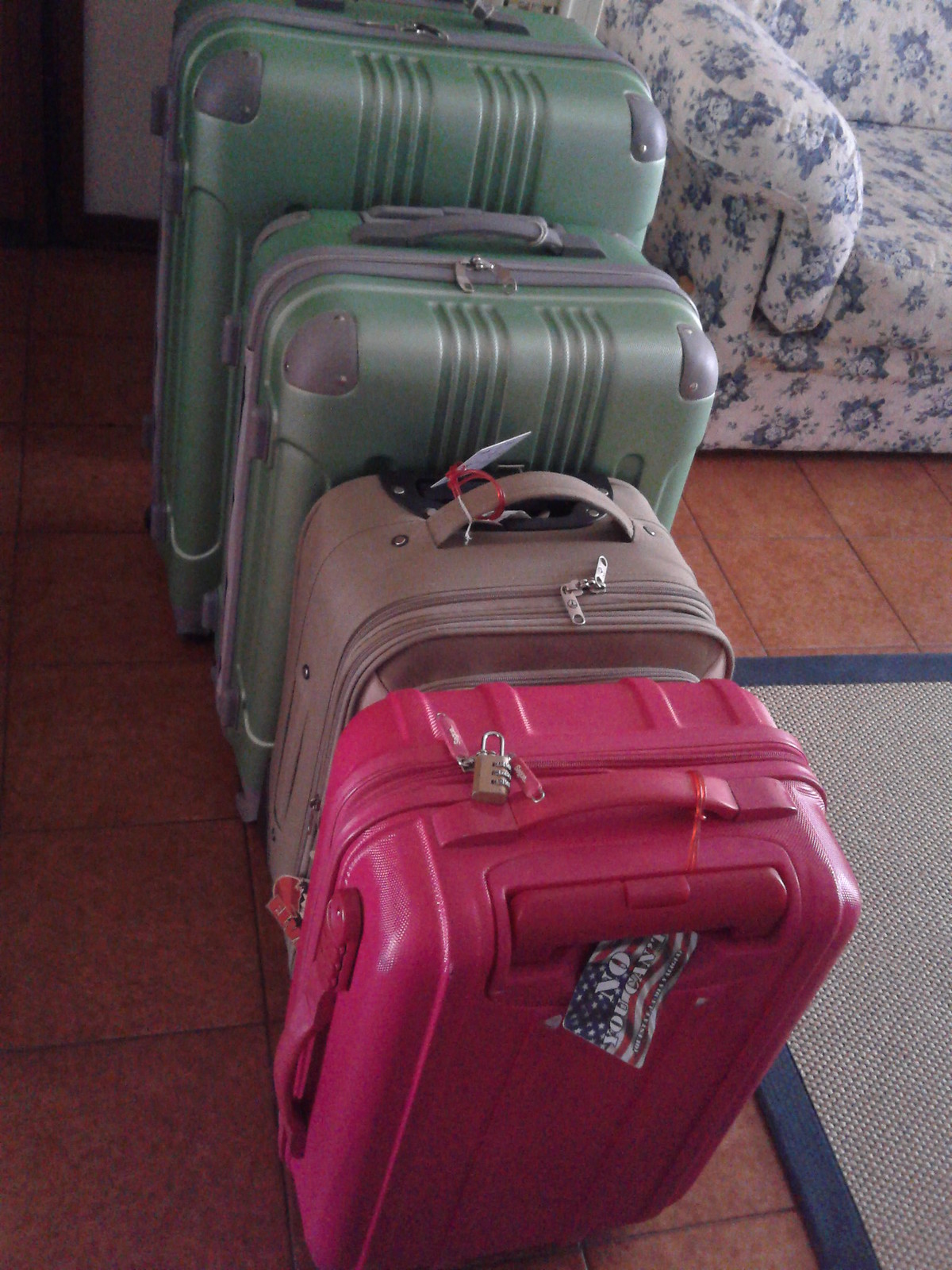This photograph, taken indoors, captures a neatly arranged row of four suitcases placed on a brown tiled floor in a living room or entryway. The suitcases are organized in a sequence from smallest to largest. At the very front is a bright pink, hard-shell suitcase adorned with a brass combination lock. An American flag tag attached to the front reads "No, you can't." Directly behind it is a tan fabric suitcase, slightly narrower and taller than the pink one. Following that is a mint green hard-shell suitcase, exhibiting gray accents on the zippers and handles. The final and largest suitcase, standing the tallest in the row, is another mint green hard-shell with gray highlights, matching the one in front but significantly larger. 

On the bottom right corner of the image, part of a jute-style rug with a dark blue trim is visible. In the top right corner, a white couch featuring a blue floral pattern peeks into the frame. The overall composition, with the descending size of suitcases and complemented by the background elements, creates a balanced and visually interesting scene.